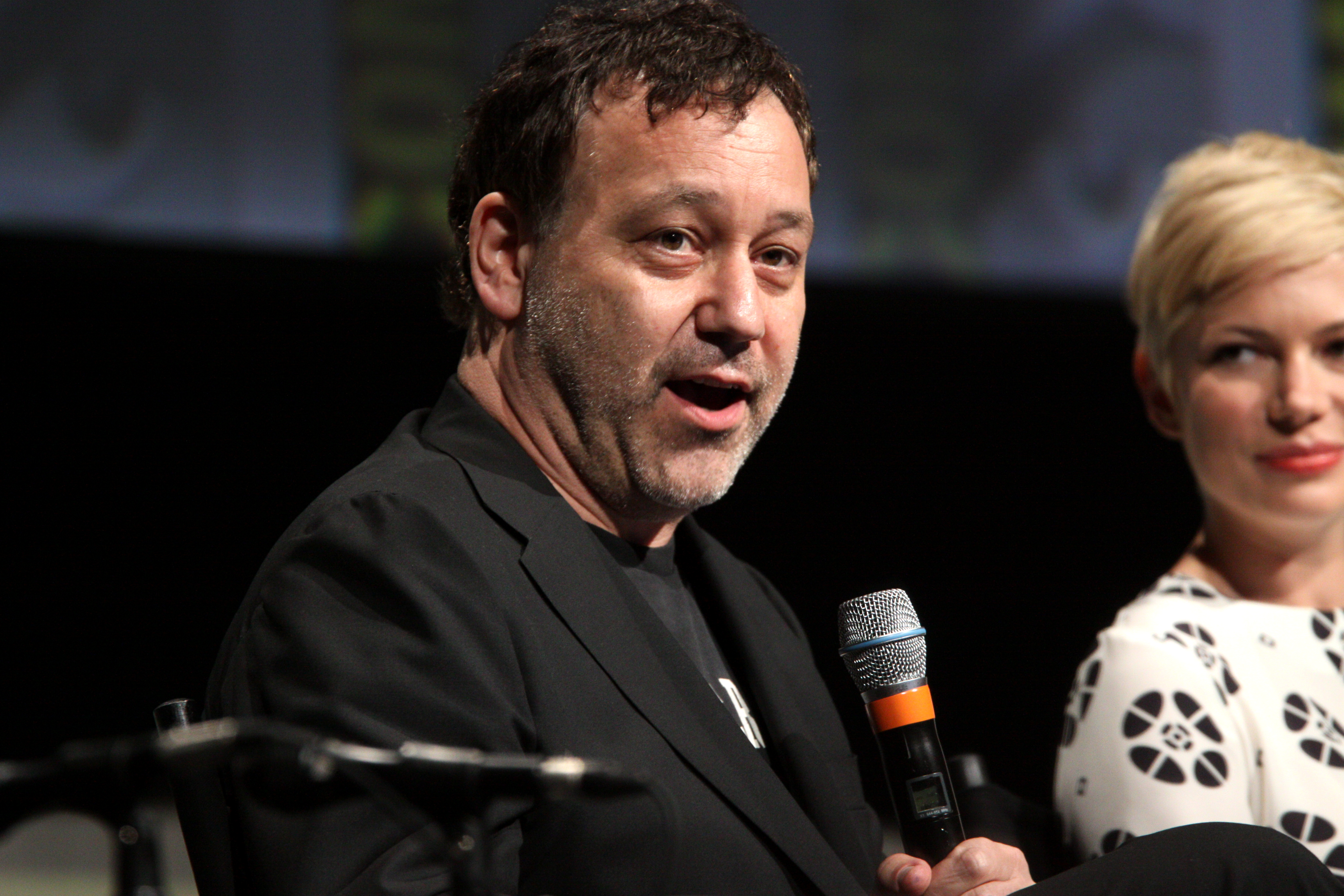In the image, a light-skinned man with dark brown hair and a slight five o'clock shadow, speckled with gray, is prominently featured. He wears a black t-shirt with a design in white letters, partially obscured, under a black blazer. The man is in the middle of speaking, holding a black microphone with a silver top and an orange strip of tape around it in his left hand. Seated next to him is a light-skinned woman with short blonde hair, gazing attentively at him. She is dressed in a white blouse adorned with black geometric shapes. The background of the image is predominantly black, adding contrast to the duo, and includes a partially visible white and yellow poster. Another microphone is noticeable in the blurred foreground.